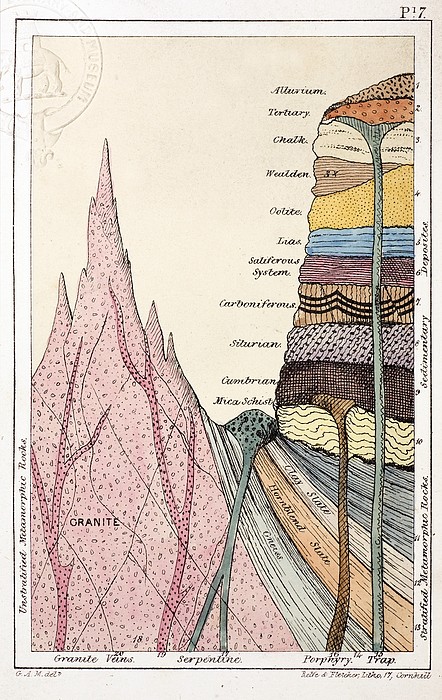The image is a detailed, hand-drawn diagram depicting various layers of soil and rock, reminiscent of an old textbook illustration. The diagram is framed with a white border and bears the label "page 17" at the top. On the left side, in distinctive pink shades with darker veins, a large granite spike is prominently labeled "GRANITE" in black, uppercase text. The right side of the image features a vertical column showing multiple sediment layers, each identified by specific labels and unique patterns such as solid colors, stripes, or polka dots to enhance visual differentiation.

From bottom to top, the layers include: Gnesis, Hornblende Slate, Clay Slate, Mica Schist, Cambrian, Silurian, Carboniferous, Siliferous System, Ironstone, Wealden, Chalk, Tertiary, and Aluminum. Each layer is depicted with distinct textures, such as the Silurian layer in a pink-peach background with black polka dots, and the Carboniferous layer in a tan color with vertical lines and a black wave pattern. The frame surrounding the diagram also contains textual labels: "Unstratified Metamorphic Rocks" on the left, "Granite Veins, Serpentine, Porphyry, Trap" at the bottom, and "Stratified Metamorphic Rocks, Sedimentary Deposits" on the right. The overall presentation is both informative and visually engaging, providing a meticulous cross-section of geological strata.